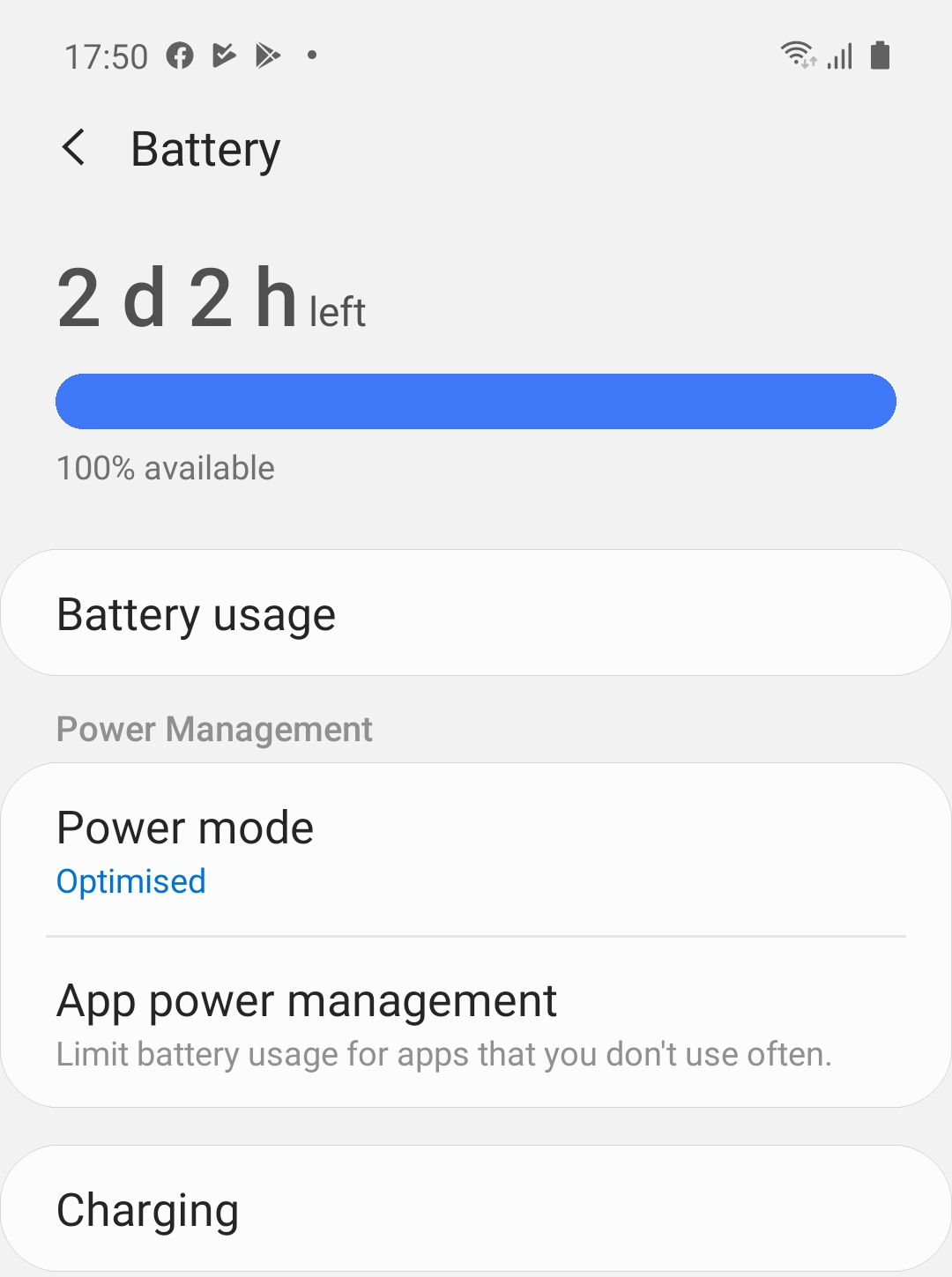This is a screenshot of the Battery Settings on a mobile device, captured at 17:50. The top left corner displays the time, alongside icons for various background apps. On the right, there are indicators for Wi-Fi signal, cellular signal, and battery life, which is at 100%. The main header reads "Battery," flanked by a back arrow on the left side. The screen shows that the battery has an estimated life of 2 days and 2 hours remaining, with 100% available. A blue power bar visually indicates full battery capacity.

Below the header, the settings are organized in different sections, each contained within white, rounded rectangles with black text. The first section, "Power Management," includes "Battery Usage" and "Power Mode" set to "Optimized." Additionally, it mentions "App Power Management," which limits battery usage for infrequently used apps. The "Charging" section is also visible. The overall color scheme is simple and minimalistic, featuring light gray and dark gray text, with the word "Optimized" highlighted in blue.